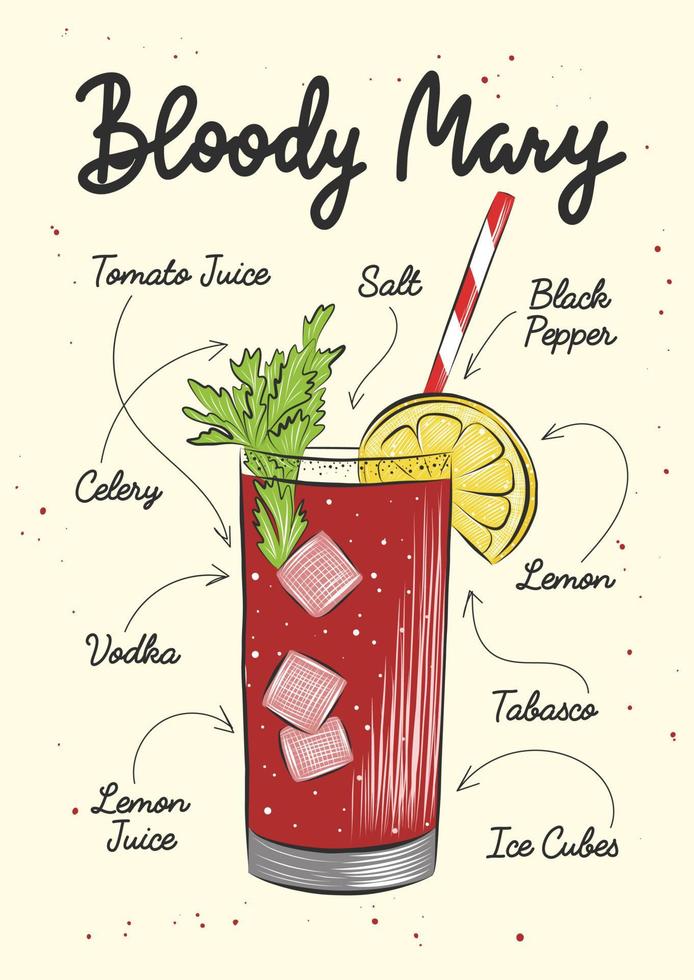The image is a detailed breakdown drawing of a Bloody Mary cocktail set against a cream-colored background. The top of the page features the hand-written, bold black cursive title "Bloody Mary." At the center of the illustration is a tall cylindrical glass filled with a vibrant red liquid, identified as tomato juice, with shining ice cubes. A green celery stalk with leaves is placed inside the glass, and a red and white striped straw rests within the drink. On the rim of the glass is a slice of lemon. The illustration includes arrows pointing to various ingredients with labels such as tomato juice, vodka, lemon juice, salt, black pepper, lemon, Tabasco, celery, and ice cubes. Scattered black and dark red dots add texture to the visual presentation. The elements are clearly marked with arrows and text that arc from the bottom left, extending over the glass and emphasizing each ingredient in this classic cocktail.